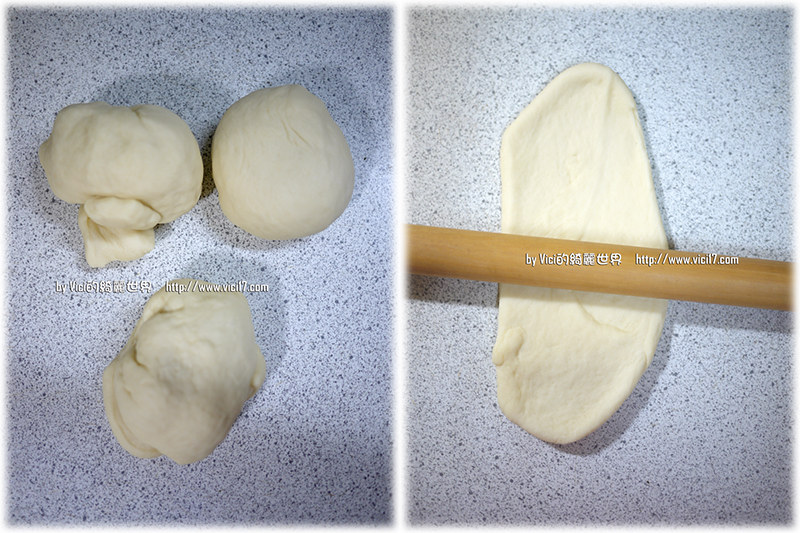The image features two vertically oriented photos side-by-side on a speckled countertop background, likely a kitchen surface. The left photo showcases three dough balls resting on the countertop, while the right photo depicts a wooden rolling pin flattening one of these dough balls into a super flat piece. Both images include a line of text running across the center, displaying a website URL: "http://www.vici17.com". Notably, the right photo also contains Chinese characters positioned above the rolling pin.